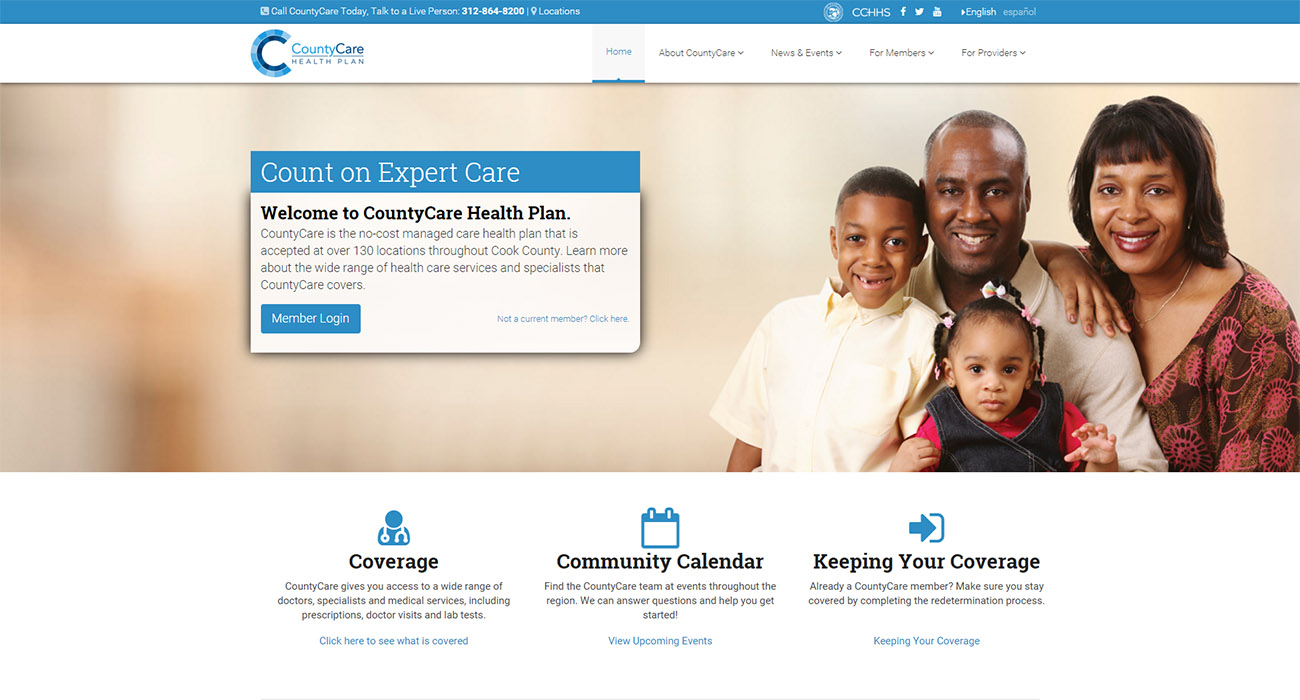Screenshot of the Country Care Health Plan website showing a family of African descent. At the top, five navigation tabs are visible: Home, About Country Care, News and Events, For Members, and For Providers. The main webpage features a heartwarming photograph of a family—a mother, father, an older boy appearing about six years old, and a young girl around two years old sitting on the father's lap. To the left, a blue bar with white text reads "Count on Expert Care," and below it, a white text box welcomes visitors with the message: "Welcome to Country Care Health Plan. Country Care is the no-cost managed health care health plan that is accepted at over 130 locations throughout Cook County." Below this text, a login button is prominently displayed.